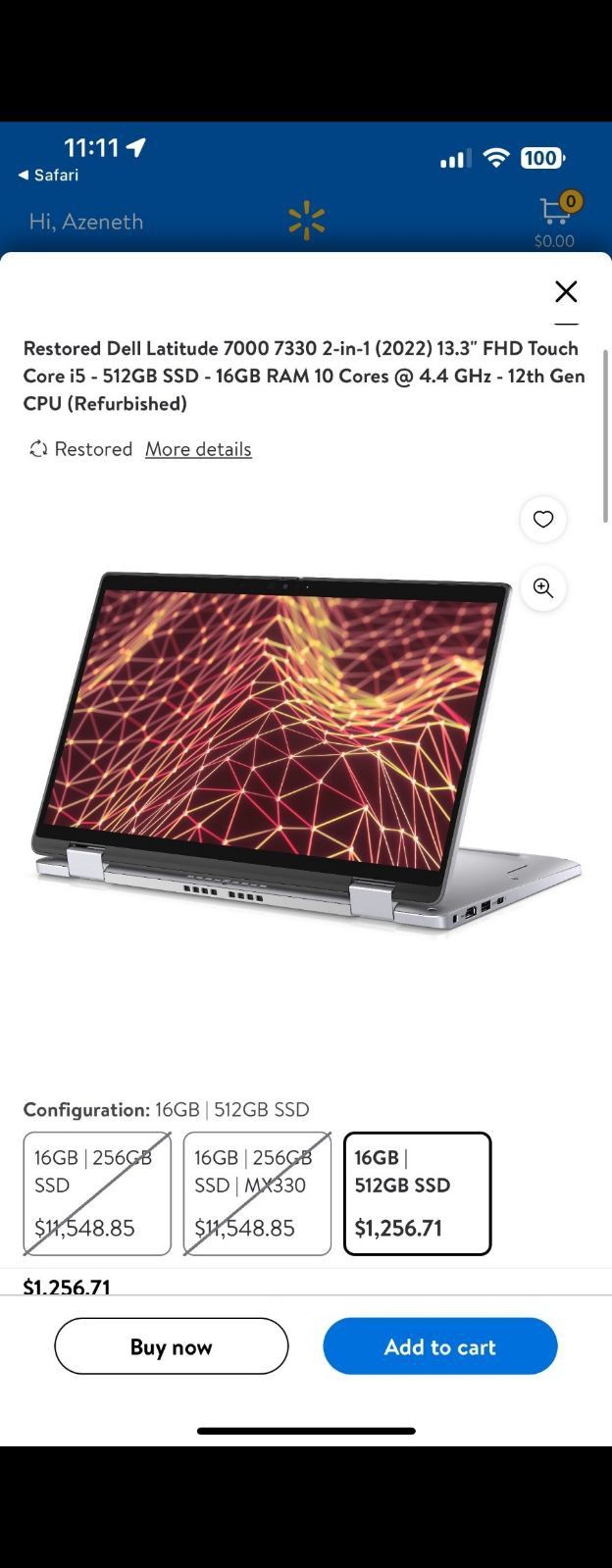In this image, we have a detailed screenshot from the Walmart app displayed on a mobile phone. The status bar at the top shows the time as 11:11, with three service bars, full Wi-Fi signal, and the battery fully charged at 100%. The app greets the user with "Hi, Azeneth" and prominently features the Walmart logo at the center.

Below, an item is listed: a "Restored Dell Latitude 7400 7330 2-in-1 (2022) 13.3-inch FHD Touchscreen." The laptop is equipped with a Core i5 processor, 512GB SSD, 16GB RAM, and a 12th generation 10-core CPU running at 4.4GHz. This is a refurbished model.

The screen includes a thumbnail image of the device, showing its versatile 2-in-1 design with the keyboard flipped backward, demonstrating its touchscreen functionality. The listing specifies that there are three options available but highlights that the only model in stock is the configuration with 16GB RAM and a 512GB SSD, priced at $1,256.71.